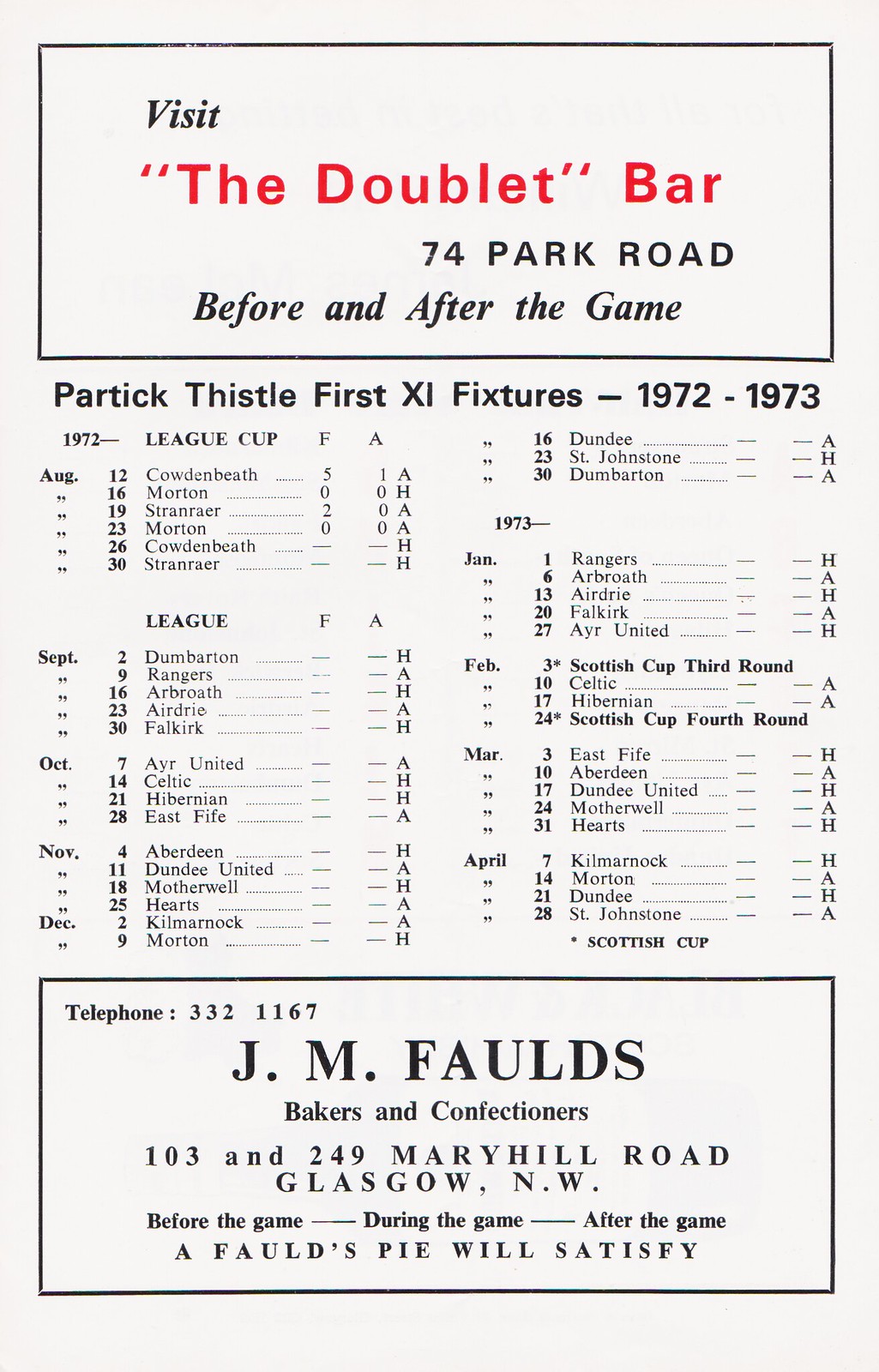This image depicts an old-style scorecard or scorebook page primarily listing the 1972-1973 first XI fixtures for Patrick Thistle. At the top, there's a promotional ad for "The Dub Lay Bar," located at 74 Park Road, highlighted in red while the rest of the text is black on a white background. Below this ad, the page details the League Cup games from August 1972 to April 1973, including various opponents and results. The page is organized in a typical layout, resembling a sheet of paper, with columns listing dates, team names, and acronyms such as F, A, and H. At the bottom, there's another advertisement for J.M. Faulds, Bakers, and Confectioners, located at 103-249 Mary Hill Road, Glasgow, Northwest, suggesting their products—emphasized by the phrase "a Fodd's Pie will satisfy"—are ideal before, during, or after the game. The overall aesthetic of the page reinforces its vintage origin, evident from the 1972-1973 seasons mentioned.